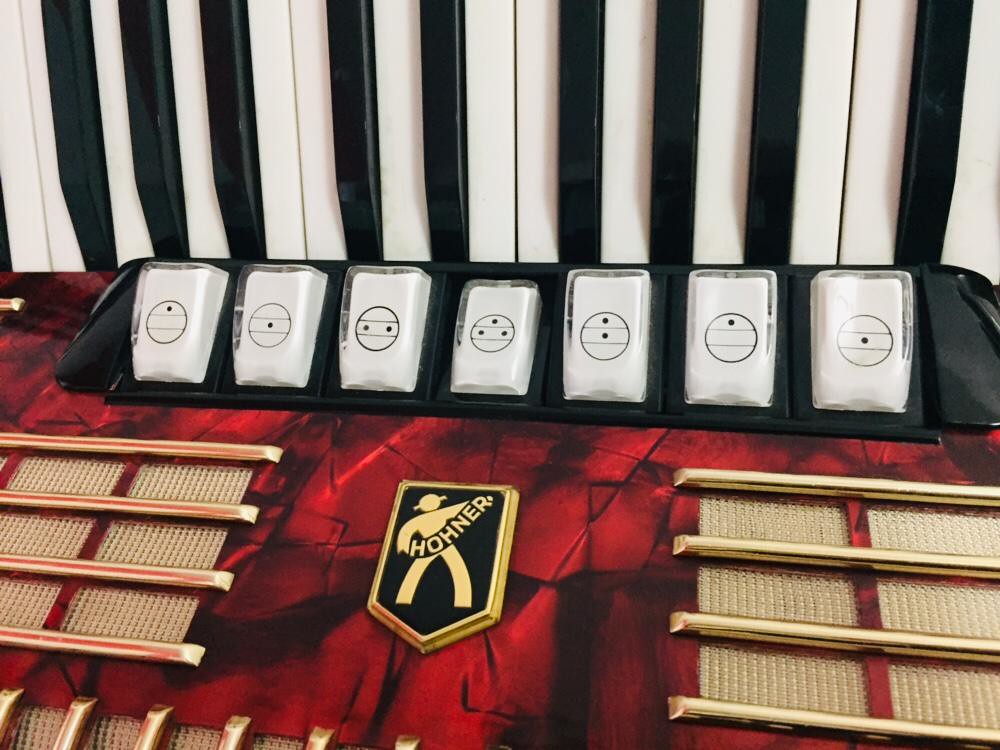This detailed close-up photograph captures a beautifully decorated Hohner accordion with a rich, reddish-black background on its case. Prominent white and black keys stretch horizontally across the top of the image. Below the keys are a series of seven white buttons, each encased in clear plastic, featuring distinct circular patterns with varying black dots. To the left and right of these buttons are golden bars set against small vent-like structures, designed to project sound. Central to the image is the Hohner logo: a gold and black emblem featuring a simplistic stick figure and the name "Hohner," H-O-H-N-E-R, shaped to mirror the contours of an accordion.